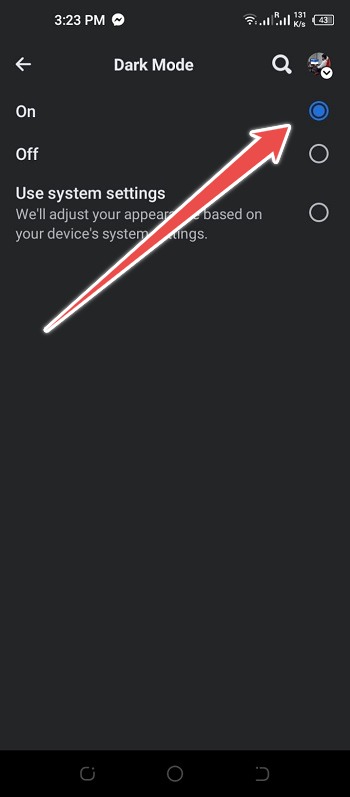Screenshot of a Smartphone Displaying Facebook Messenger Dark Mode Settings

The screenshot originates from a smartphone interface, captured at 3:23 PM. The top-left corner displays the time along with an icon resembling a graph with a line through it. A Facebook Messenger notification is also present at the top. On the top-right, the screen shows a Wi-Fi icon with three-quarters signal strength, followed by two cellular signal indicators—one with three out of four bars and the other with a full four-bar signal. The data transfer rate is indicated as 131k/s (kilobytes per second). Finishing the top bar, the battery level is shown at 43%.

Centered beneath the status bar, the title "Dark Mode" is prominently displayed in bold white text. To the left of this text is a white arrow, and to the right, a magnifying glass icon and a small profile picture of a person seated at a computer.

The subsequent section includes two options for dark mode settings: "On" and "Off." The "On" option is currently enabled as indicated by a blue-checked circle, emphasized by a long red arrow pointing toward it. The "Off" option is unchecked. 

At the bottom, in bold white text, it reads "Use system settings," followed by a grey text description: "We'll adjust your appearance based on your device's system settings." This descriptive text is partially obscured by the red arrow.